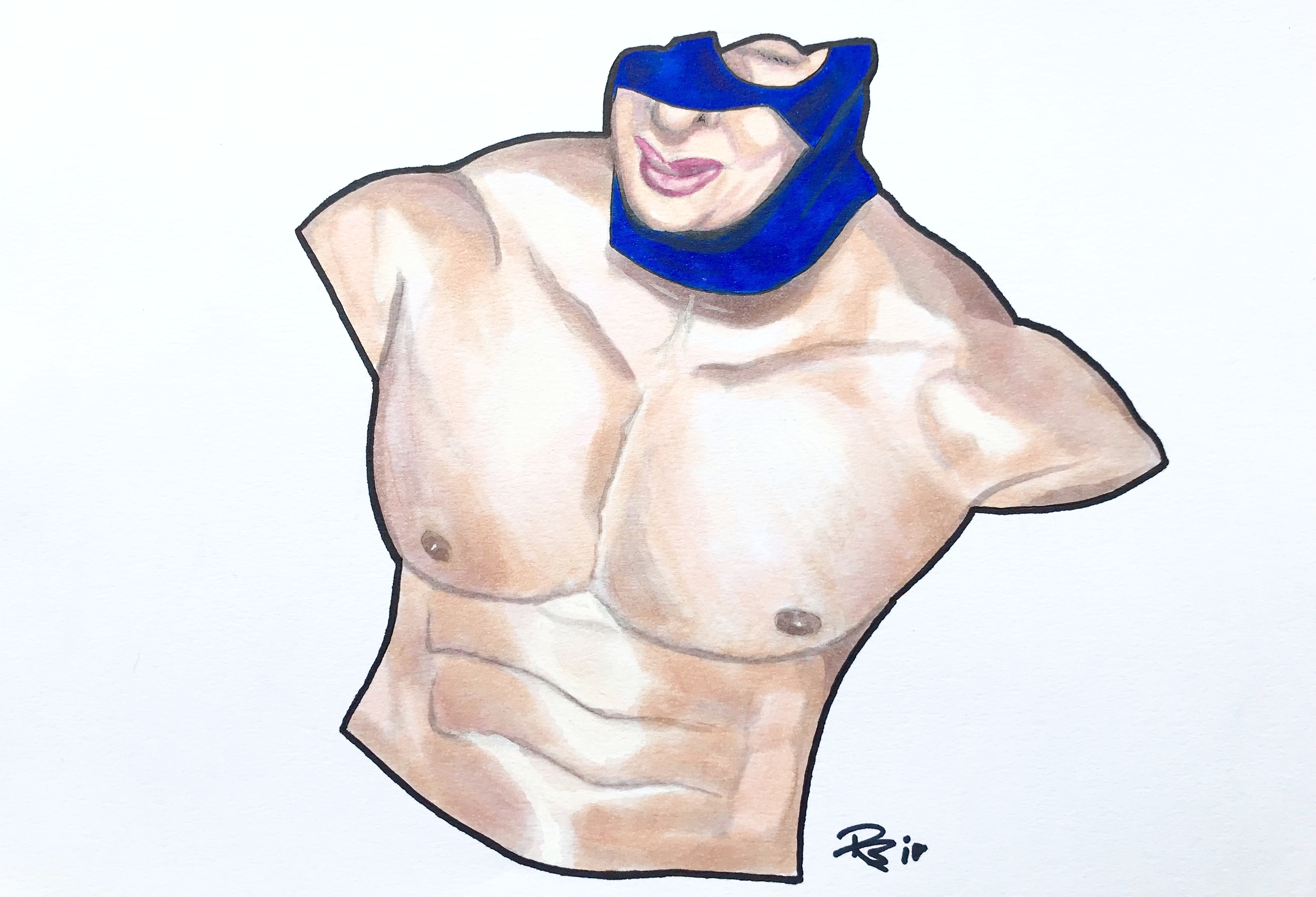This image features an intricately detailed, colored pencil drawing on a faintly blue-tinted background that is almost white. The artwork depicts the muscular torso of a man with well-defined pectoral muscles and a visible six-pack abs, but his arms have been omitted, and the drawing ends just below his chest. The man's face is partially visible; it is obscured by a blue mask similar to those worn in Mexican wrestling, revealing only his left eye and his nose. His mouth is open, exposing his pink lips and tongue. The top of his head and his right eye are cut off from the frame. Signed by the initials "RBID" located underneath the left nipple, this image uses a palette of black, white, brown, tan, blue, and pink to create a striking visual effect. The exaggerated musculature and the partial depiction of the figure suggest that it might be an art piece, potentially part of a book or another illustrative medium.